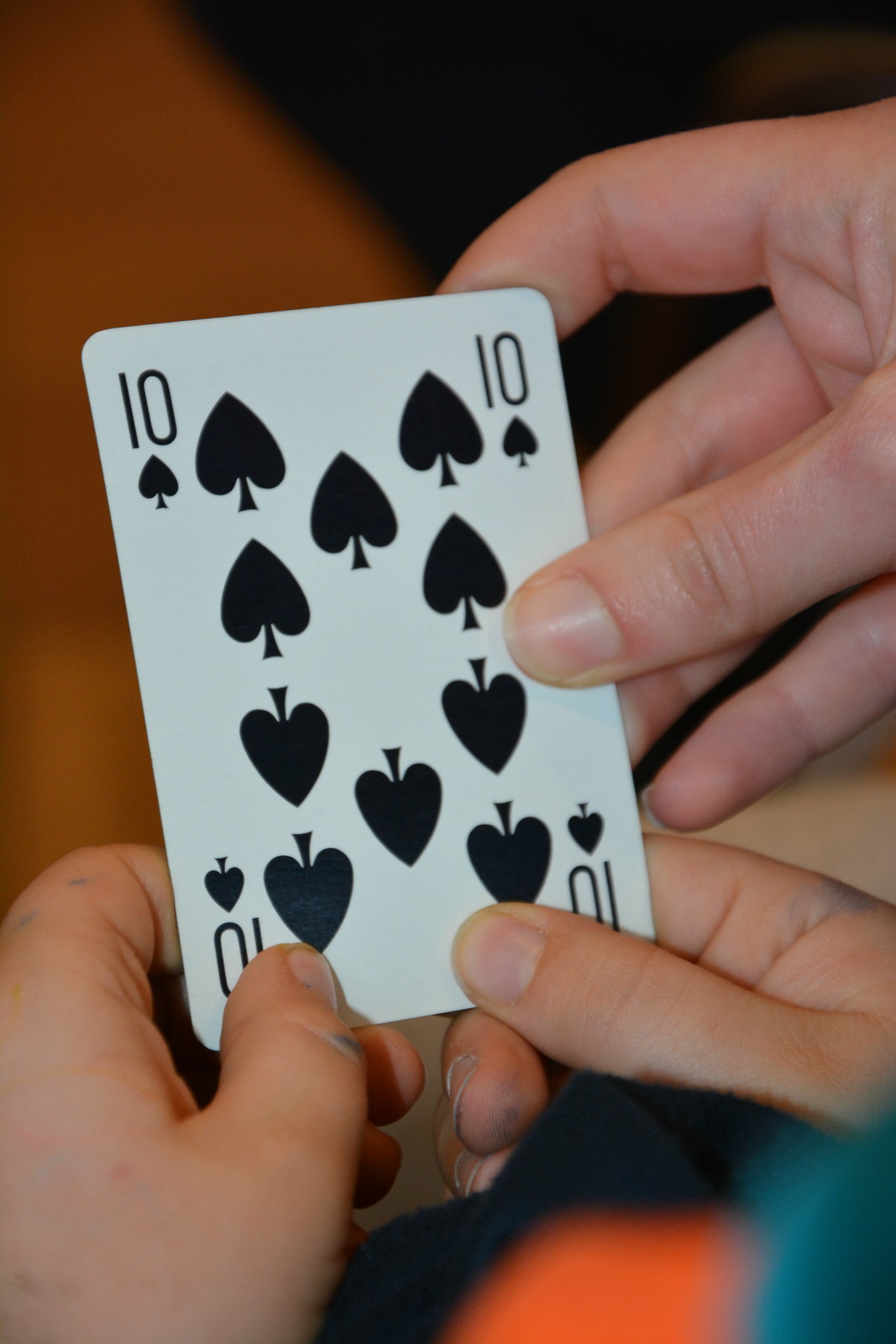In the image, three hands are holding a Ten of Spades playing card against a white background. The card, prominently displayed, features the number ten and black spade symbols in all four corners. Two hands positioned at the bottom of the card, one on the left and the other on the right, grip the card carefully. These hands are noticeably marked with blue or black smudges, possibly from a marker, indicating they are quite dirty. In contrast, the third hand, which holds the card from the middle right side with the thumb placed centrally, appears freshly manicured and clean. The camera has focused sharply on the hands and the card, rendering the background elements blurry and indistinguishable.